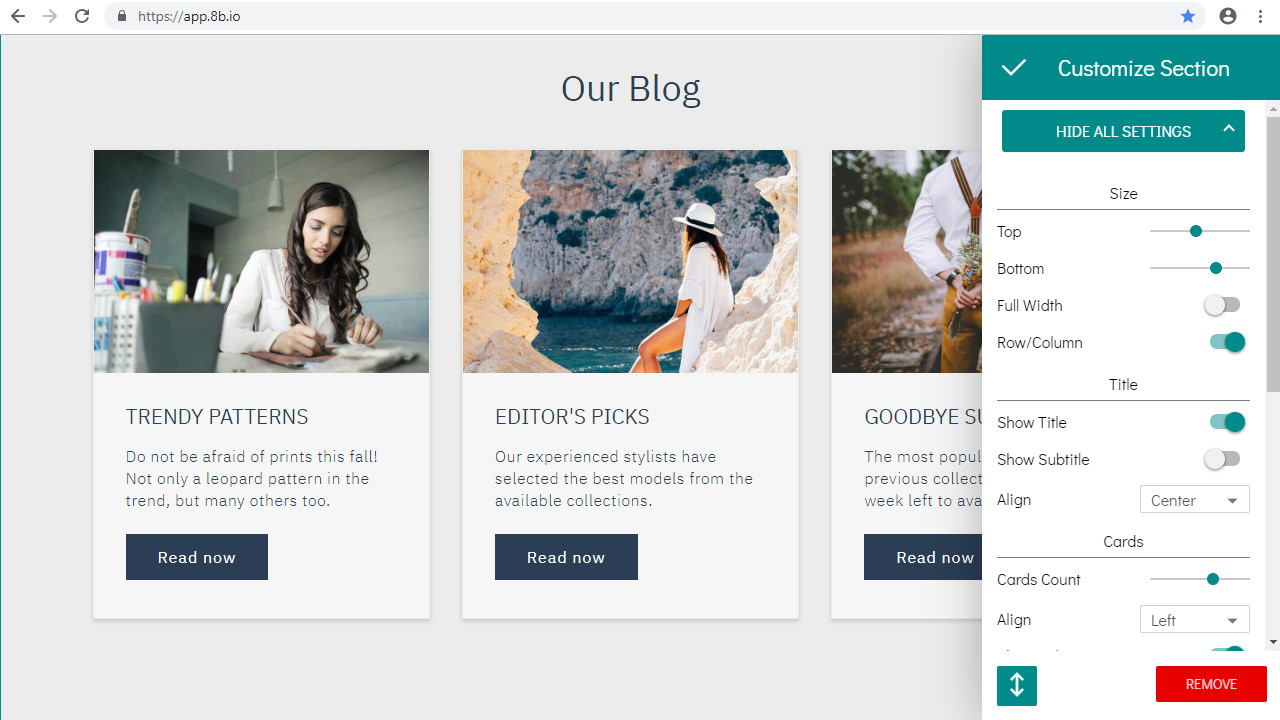This image is a screenshot of a digital device, possibly a monitor or tablet, displaying a webpage from app.8b.io titled "Our Blog." The page features three horizontally arranged panels, each with a unique title and accompanying image. 

1. The first panel, named "Trendy Patterns," shows a woman writing in a notebook with a pen, capturing a moment of thoughtful creativity.
2. The second panel, titled "Editor's Pick," features an outdoor scene of a woman wearing a white hat and a white bathing suit cover-up, suggesting a casual and relaxed setting.
3. The third panel, titled "Goodbye Something," depicts a man holding a bouquet of flowers behind his back, hinting at a poignant or romantic gesture.

On the far right of the screen, there is a teal-colored pop-up labeled "Custom Selections," presenting various customizable options for the user.